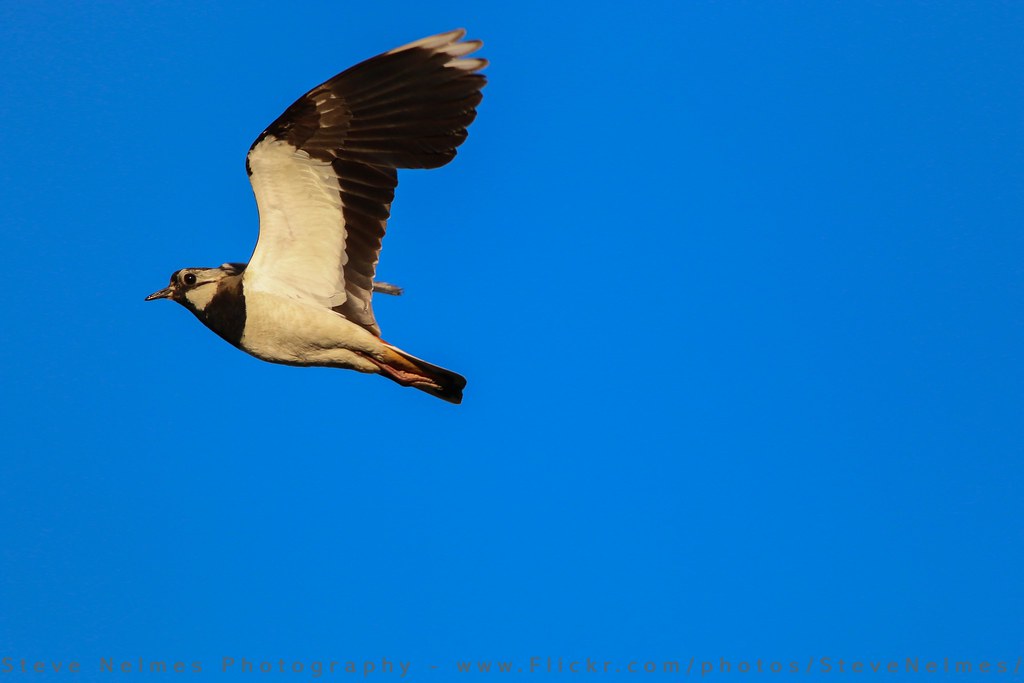This horizontal, realistic photograph by Steve Niemes Photography captures a black and white bird soaring against a bright blue sky, positioned slightly to the left of the center. The bird, with its wings fully stretched out, showcases a striking pattern: its black neck contrasts sharply with its white face and black beak. The underbelly is white, with black wings accented by white tips and white patches closer to the body. The bird's feet are tucked in and are a pale pinkish-orange color. The serene, uncluttered background emphasizes the elegance and beauty of the bird in mid-flight, highlighting the simplicity and natural grace of the moment. No text is present in the image itself, and the overall tone is one of tranquil realism, as if the photograph was captured spontaneously.